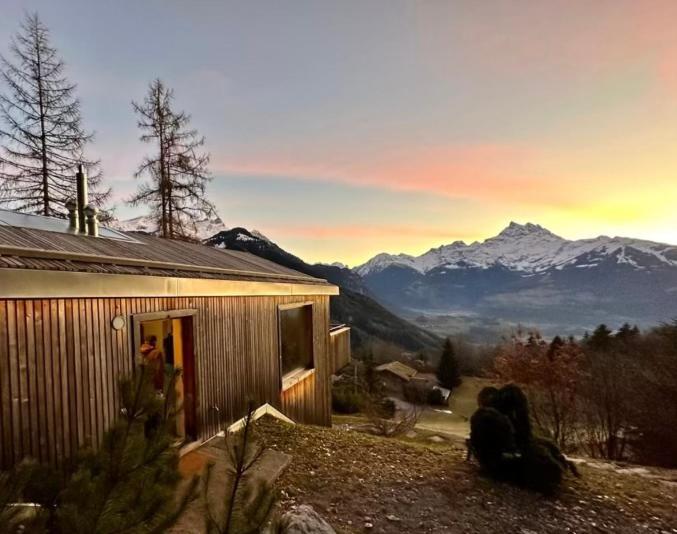This photo captures a serene, rural mountain cabin scene at sunset. The cabin, constructed from vertical wooden panels, stands elevated on a rocky incline, with the left side showcasing a door, multiple windows, and a balcony. The setting sun casts an orange hue on the snowy distant mountains and reveals leafless trees, suggesting it is winter. The valley below is filled with additional trees and bushes, while branches resembling those from Christmas trees lie in the foreground. The sky is a blend of wispy orange clouds and patches of blue. In the bottom middle of the image, a large rock is visible, and there is a person standing at the sliding door, further enhancing the tranquil life in this secluded setting.